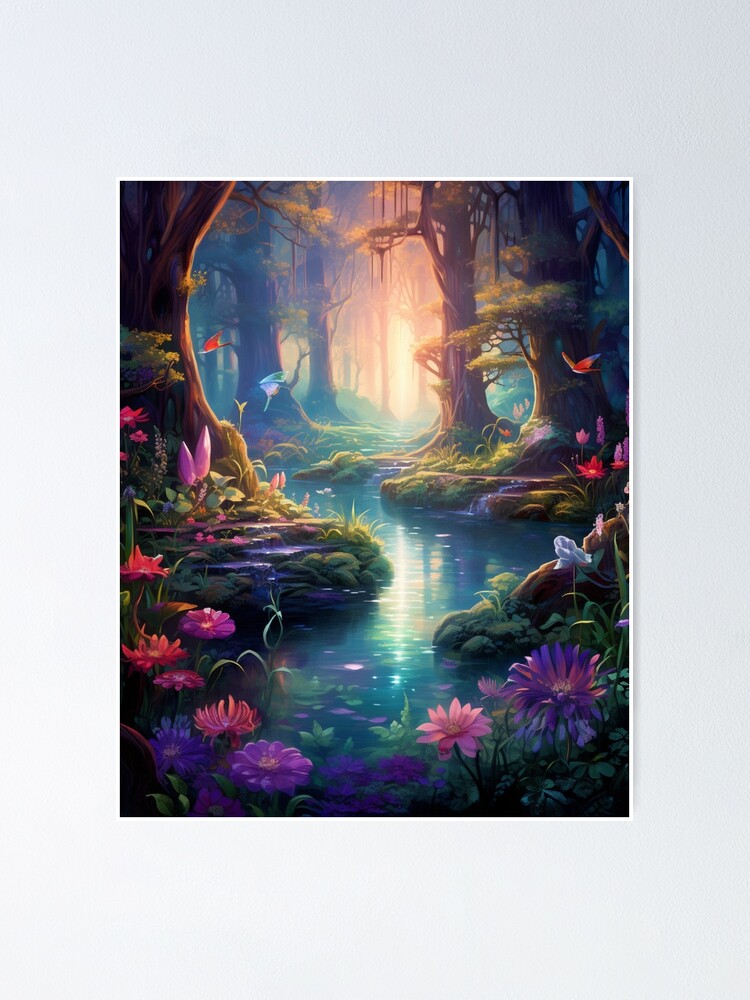This vibrant and fantastical painting depicts a serene brook winding through an enchanting forest. The brook is a brilliant deep blue, sparkling as sunlight filters through the dense canopy. The edges of the brook are adorned with old growth trees, draped with vines and moss, creating a tunnel-like effect. The forest floor and brook banks burst with colorful flowers in shades of purple, pink, and red. Various birds, including a blue bird and two red birds, flit among the trees. Amidst the natural beauty, mythical elements emerge: a large ostrich-like figure looms in the background, and a mysterious blue object with glasses and a knit cap adds a whimsical touch. Glittering in the distance, a dazzling sunrise or sunset bathes the scene in ethereal light, enhancing its fairy tale ambiance. The overall effect is a bold, fantastical scene where vivid colors—greens, magentas, and teals—transform the natural setting into a dreamlike landscape.